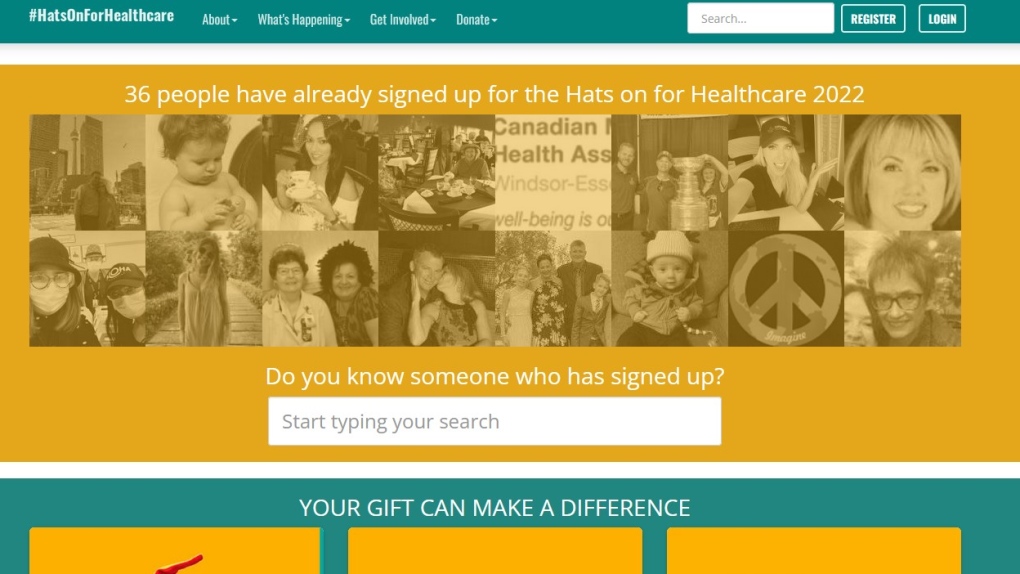The image is a screenshot of a webpage, dominated by a dark teal-colored bar at the top. In the top-left corner of this bar is the phrase "#HatsOnForHealthCare," with each word capitalized. The bar also contains navigation options such as "What's Happening," "Get Involved," and "Donate." On the right side, there is a white search bar followed by two buttons: "Register" and "Log In."

Below this, a thin white horizontal strip runs across the page. Directly beneath it, there is a large golden box. At the top of this box, in white text, it states, "36 people have already signed up for the Hats On for Health Care 2022." The box contains a montage of various images, all filtered with a golden hue. The images include diverse scenes such as a baby, a woman at a tea party, a peace sign, a blonde woman, a couple, two friends, individuals wearing white masks, a woman on a boardwalk, another baby in a white hat, people posing with a trophy, and others, including shots of a party and a duo in front of what seems to be the Space Needle in Seattle.

Below the montage, white text asks, "Do you know someone who has signed up?" followed by a white search bar that prompts, "Start typing your search." Another thin white strip demarcates the end of this section. Finally, at the bottom of the page, a blue box features white capital letters that read: "YOUR GIFT CAN MAKE A DIFFERENCE."